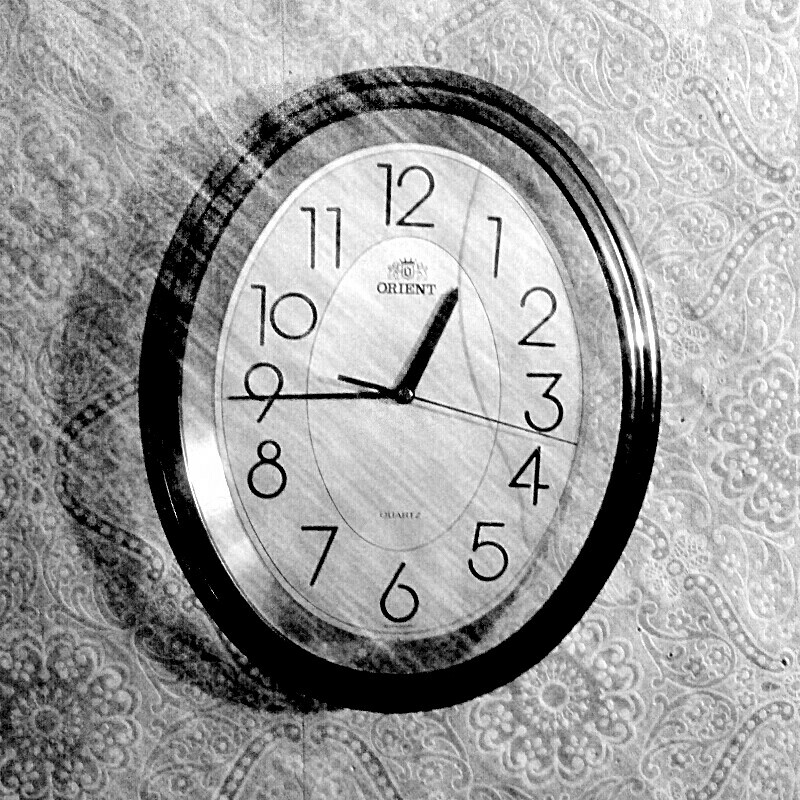Photographed in black and white, this image captures a classic wall clock mounted against an intricately patterned vintage wallpaper. The wallpaper exudes an old-fashioned charm with its elaborate, possibly floral motifs. The clock itself boasts a traditional design with a black circular frame encompassing a white background. The black numerals are displayed in a conventional serif font, accentuating the clock's timeless aesthetic. Positioned at the top center of the clock face is the branded logo, "Orient." The photograph was taken at approximately 12:45, as indicated by the clock hands. The monochromatic theme may have been achieved through digital alteration, enhancing the overall nostalgic and retro ambiance of the scene.